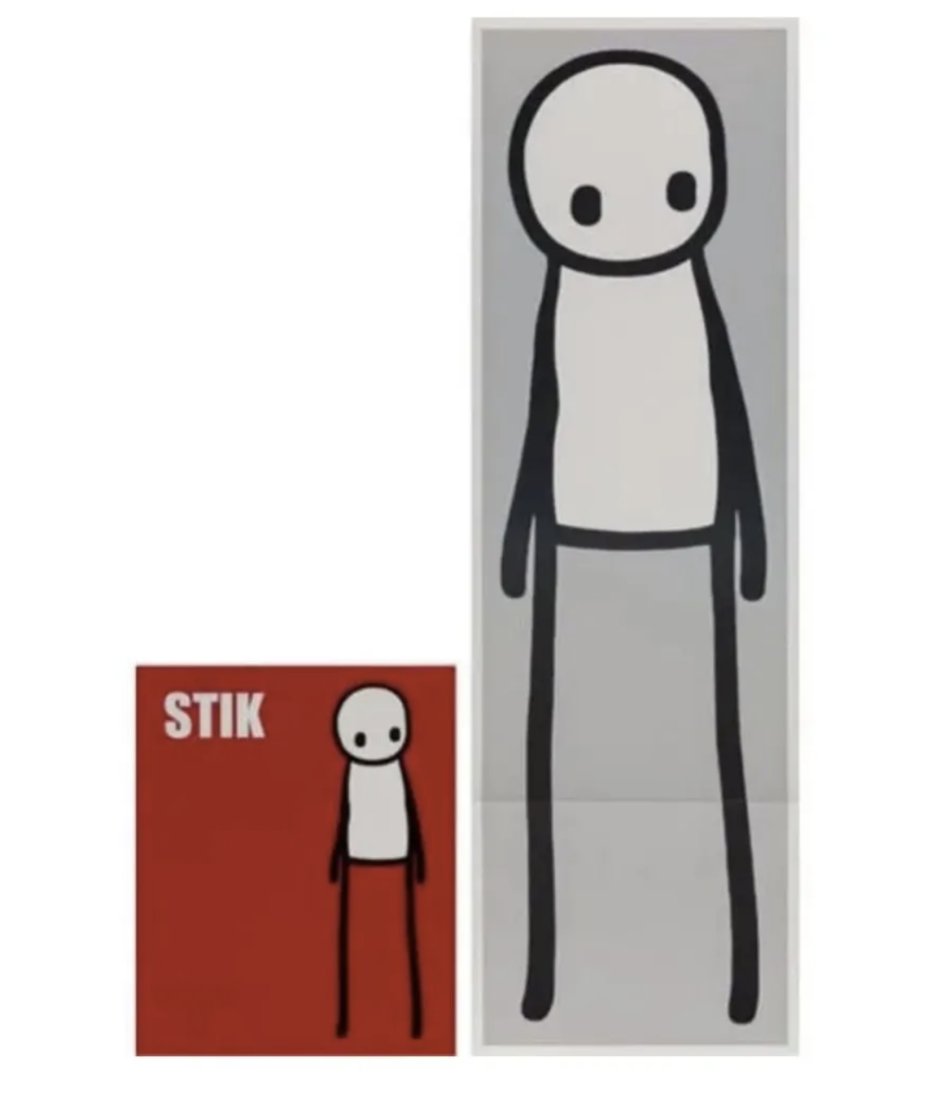In this dual-image artwork, two posters are positioned side by side. The poster on the left is a small red square featuring a minimalist stick figure drawn in black with a white face and torso. This figure, gazing down and to the right, has thin stick arms and legs and occupies the right side of the red square. In the upper left corner of this red poster, the white text "S-T-I-K" is prominently displayed. To the right, there is a larger, vertical rectangular poster in light gray, showcasing a nearly identical stick figure, taller and still looking down to the right. This gray poster features a darker gray background with a light gray trim along its edges. A horizontal crease mark is visible a couple of inches from the bottom, aligning with the figure's knees, giving the impression that the poster has been folded. The artistic style appears simplistic and digitally rendered, evocative of basic graphics software like Microsoft Paint.